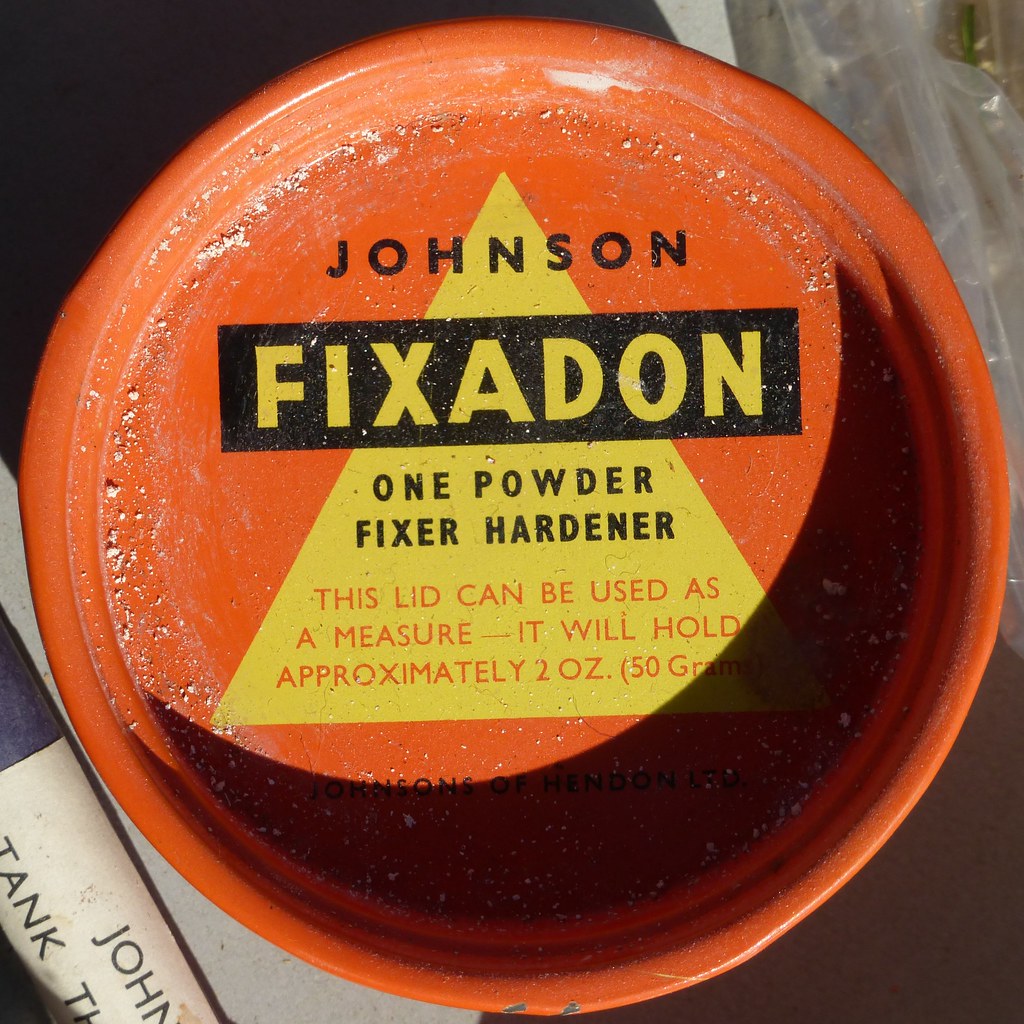This is a detailed photograph featuring the worn lid of an orange container against a black and brown background. The lid is prominently displayed in the center of the image, and it has a wide brim. In the middle of the lid, there's a yellow triangle with various inscriptions. At the top of this triangle, in black letters, it reads "Johnson." Cutting through the triangle, the capital letters "H," "N," and "S" are present. Below these letters, within a black rectangle, the word “Fixadon” is written in larger yellow text. Underneath, additional black text states "One Powder Fixer Hardener." Further down, in red letters, it specifies, "This lid can be used as a measure. It will hold approximately 2 ounces, 50 grams." Surrounding the lid, there's some white, powdery material partially obscuring more text, but the words "Johnsons of Hendon" are still discernible. To the left of the lid, a folded newspaper with the partial text "John Tank" and plastic covering can be seen, while the upper right corner of the image shows the plastic slightly wrinkled.